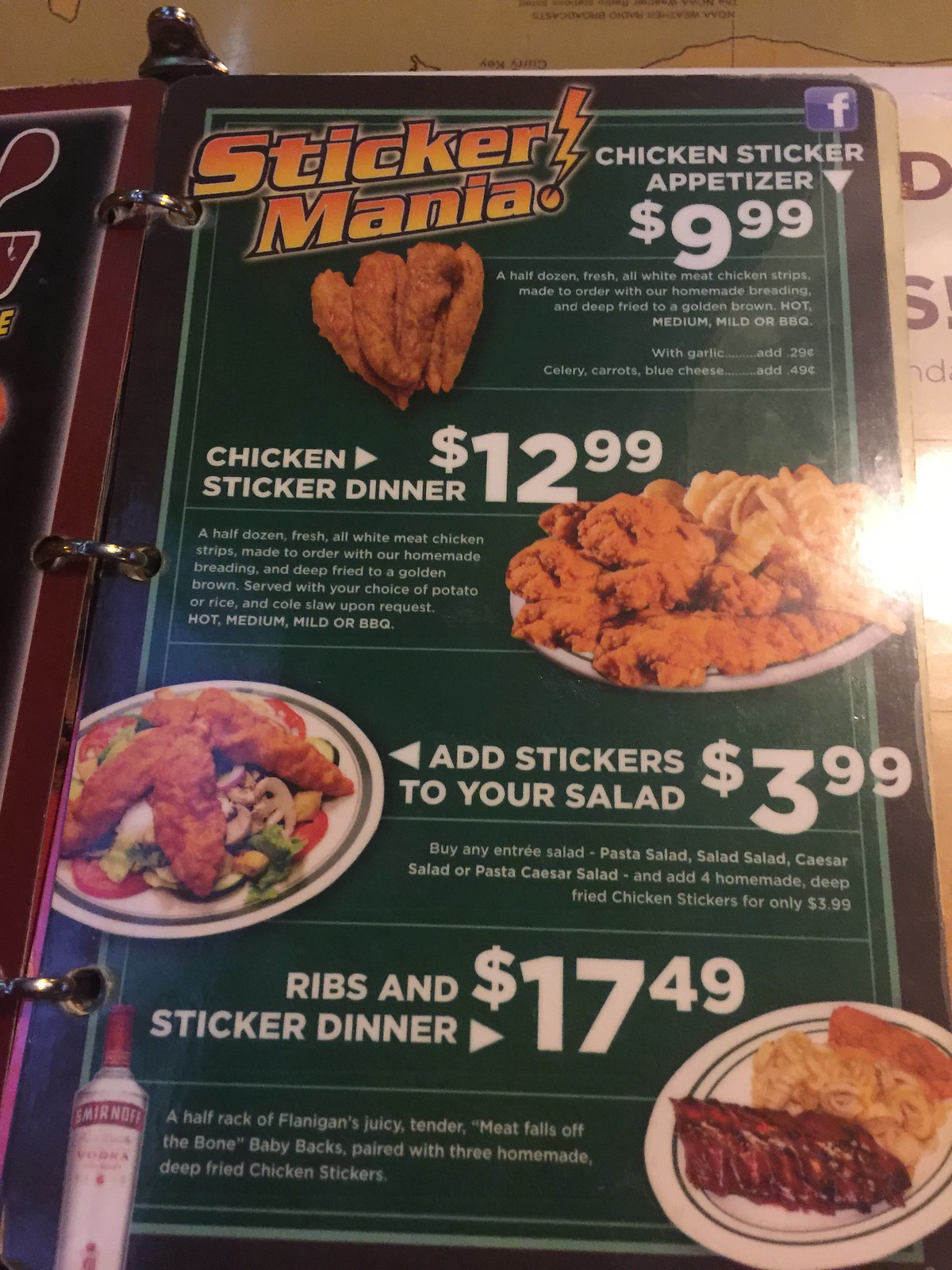The photograph showcases a unique, vintage-style menu designed like an old school notebook, complete with a metal clip mechanism at the top, allowing pages to be turned or swapped out. The main page of the menu features a vibrant green background. In the upper left-hand corner, bold text in yellow and orange reads "Sticker Mania," accompanied by a lightning bolt acting as an exclamation point.

To the right of this logo, in crisp white font, the item "Chicken Sticker Appetizer" is listed, priced at $9.99. Just above this text, there’s a small Facebook icon. Below the item title, a description in white font briefly explains what the appetizer entails. Adjacent to this, on the left, there’s a tantalizing photograph depicting four Chicken Sticker Appetizers.

Beneath this section, "Chicken Sticker Dinner" is displayed in white font with a price tag of $12.99. A descriptive blurb in a smaller white font elaborates on the dish’s components. To the right, there’s an image showcasing a plate of the Chicken Sticker Dinner.

As you move down the menu, another item is presented: "Add Stickers to Your Salad for $3.99," written in white font on the right side of the page. On the left, there's an appetizing picture of a salad adorned with three stickers.

Finally, at the bottom of the menu, "Ribs and Sticker Dinner" is listed at $17.49, accompanied by a photograph on the right illustrating the dish, making it a comprehensive visual and textual description of the menu's offerings.